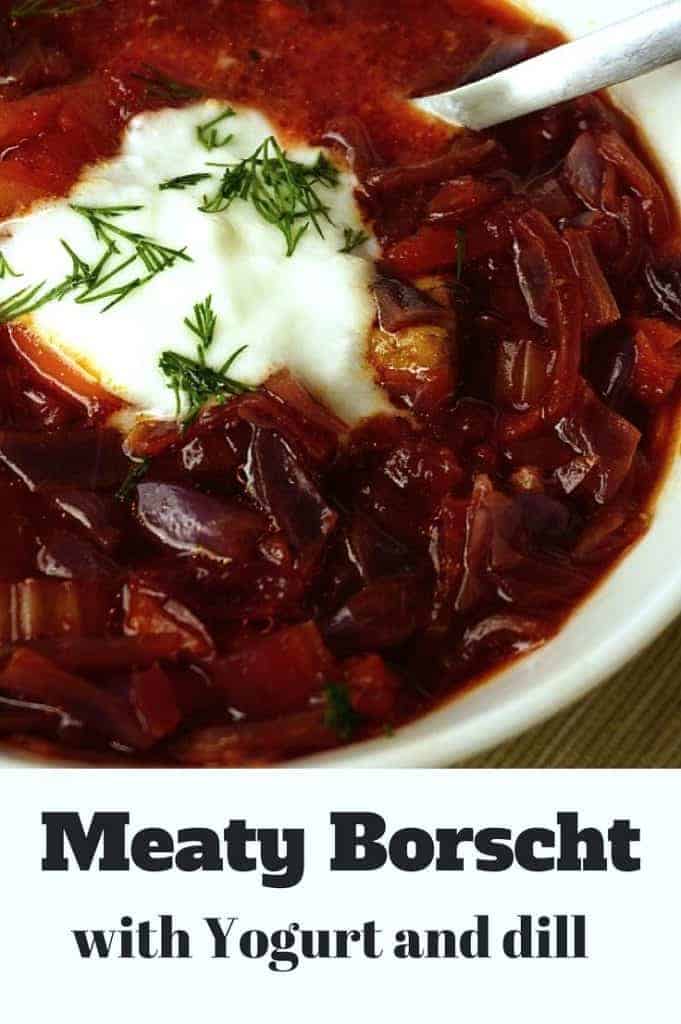This image features a close-up of a bowl of Meaty Borscht, as indicated by the black text at the bottom which states "Meaty Borscht" in large letters, followed by the description "with yogurt and dill" in smaller letters. The borscht, a hearty soup, is presented in a white bowl situated on a greenish-brown lined table setting. A silver spoon is deeply immersed in the dark reddish-brown broth, with only the handle visible above the surface. The borscht appears richly textured, with hints of tomato, pepper, or meat pieces discernible within the vibrant red mixture. At the center of this appetizing dish is a dollop of white yogurt, topped with a sprinkle of fresh green dill, adding a touch of color contrast and garnish. The overall presentation suggests a promotional image, possibly for a recipe or a restaurant menu, highlighting the delicious and visually appealing nature of this meaty borscht with yogurt and dill.